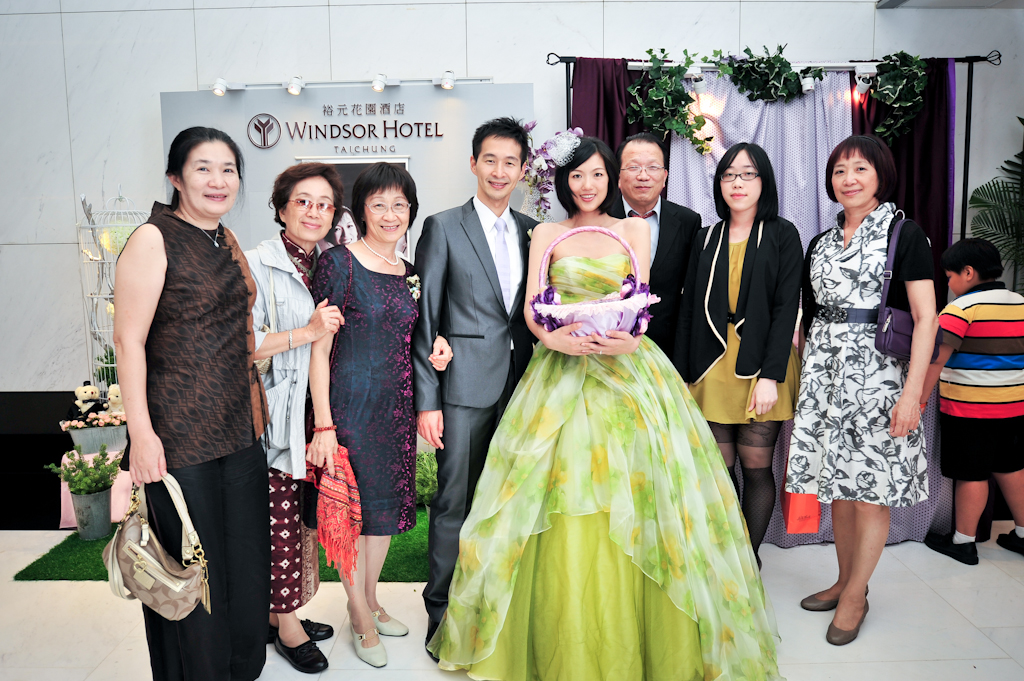The photograph is a vibrant full-color image taken indoors at a formal event, likely a wedding, held at the Windsor Hotel Taichung. The setting features pristine white walls and tiled flooring, emphasizing the elegance of the venue. Centered in the image is a group of nine people, mostly adults, with a younger boy positioned on the far right, noticeable by his multicolored shirt and his back turned toward the camera. 

Dominating the background is a lit-up banner with the text "Windsor Hotel" along with some Asian writing, which adds a touch of cultural context. There are also white and dark curtains on the right adorned with hanging plants, contributing to the sophisticated decor. The attendees, who are looking directly at the camera and smiling, include a young woman in an elegant, sleeveless green dress holding a basket, suggesting a role of significance in the event, possibly as a bridesmaid. Next to her is a young man in a shiny gray suit, complementing her formal attire.

To the left of this couple stand three older women, while to her right are an older man and two other women, presenting a diverse age range and hinting at family relations or close friendship. The image exhibits a rich palette of colors including white, green, tan, purple, pink, dark blue, light green, black, and yellow, which enhances the overall festive and joyous atmosphere of the occasion.